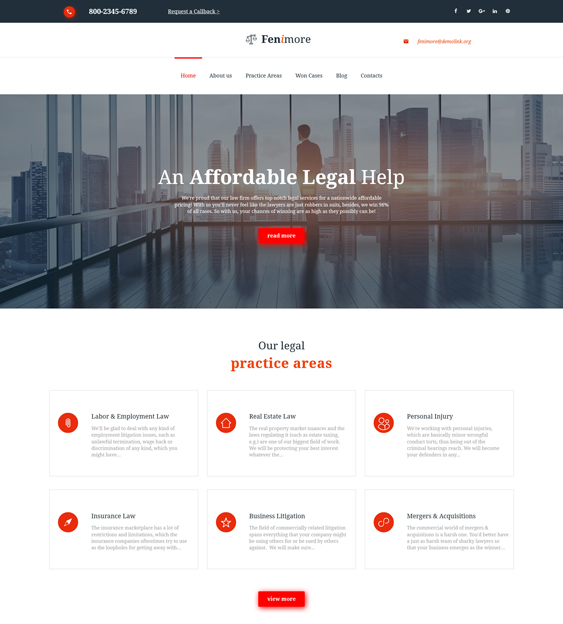Certainly! Here's a detailed and cleaned-up caption for the image:

---

The screenshot features a clean white background with multiple icons and text elements:

- At the top of the image is a red circle containing a white phone icon, symbolizing contact information.
- To the left, social media icons are arrayed, including Facebook, Twitter, Gmail (denoted by a "G" for Google), and LinkedIn (denoted by "IN").
- The name "Fenny Moore" is displayed prominently, with "Fen" in capital letters and an orange "I".
- Beneath the name, navigation options are listed in orange: "Home," "About Us," "Practice Areas," "Win Careers," "Blog," and "Contact Us."
- A tagline, "Affordable Legal Help," is displayed on the image, highlighting the service offered.
- In the main visual, a man is standing in an office, gazing out of a window at a city skyline.
- Below the image, a red rectangle with white text reads "Our Legal Practice Areas."
- There are six orange rectangles listed below this, each detailing a specific legal practice area:
  1. Labor and Employment Law
  2. Real Estate Law
  3. Personal Injury
  4. Insurance Law
  5. Business Litigations

The overall design aims to convey comprehensive legal services provided by the entity.